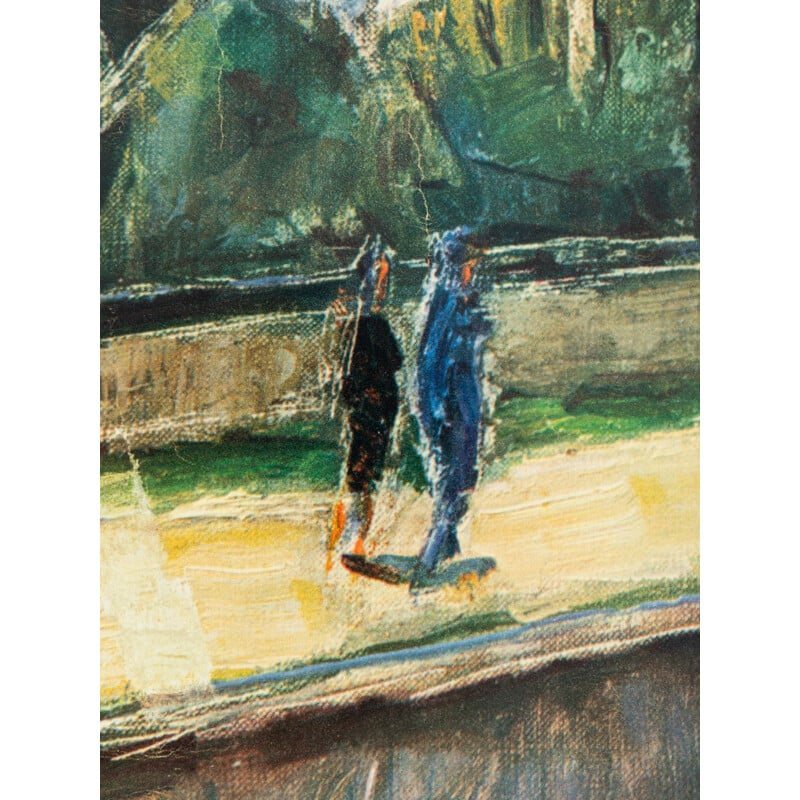This detailed and abstract painting, possibly done on canvas or digitally rendered in watercolor, depicts two human figures walking away from the viewer on a sand or dirt path. The upper portion of the image is a blend of green, blue, and yellow strokes suggesting a forest backdrop, though its abstract nature leaves the details ambiguous. Below this, a long concrete wall with a black line at the top is tinged with green, hinting at moss growth. At the base of the wall is a narrow strip of green grass, roughly two feet wide. The dirt path, a bright yellow and cream color, extends from this grassy verge. The figure on the right is dressed in blue, while the figure on the left, potentially in a skirt or dress ending above the knees, is dressed in black. Both figures may be wearing headpieces or scarves, contributing to the overall impression of a tranquil stroll along a stream path.